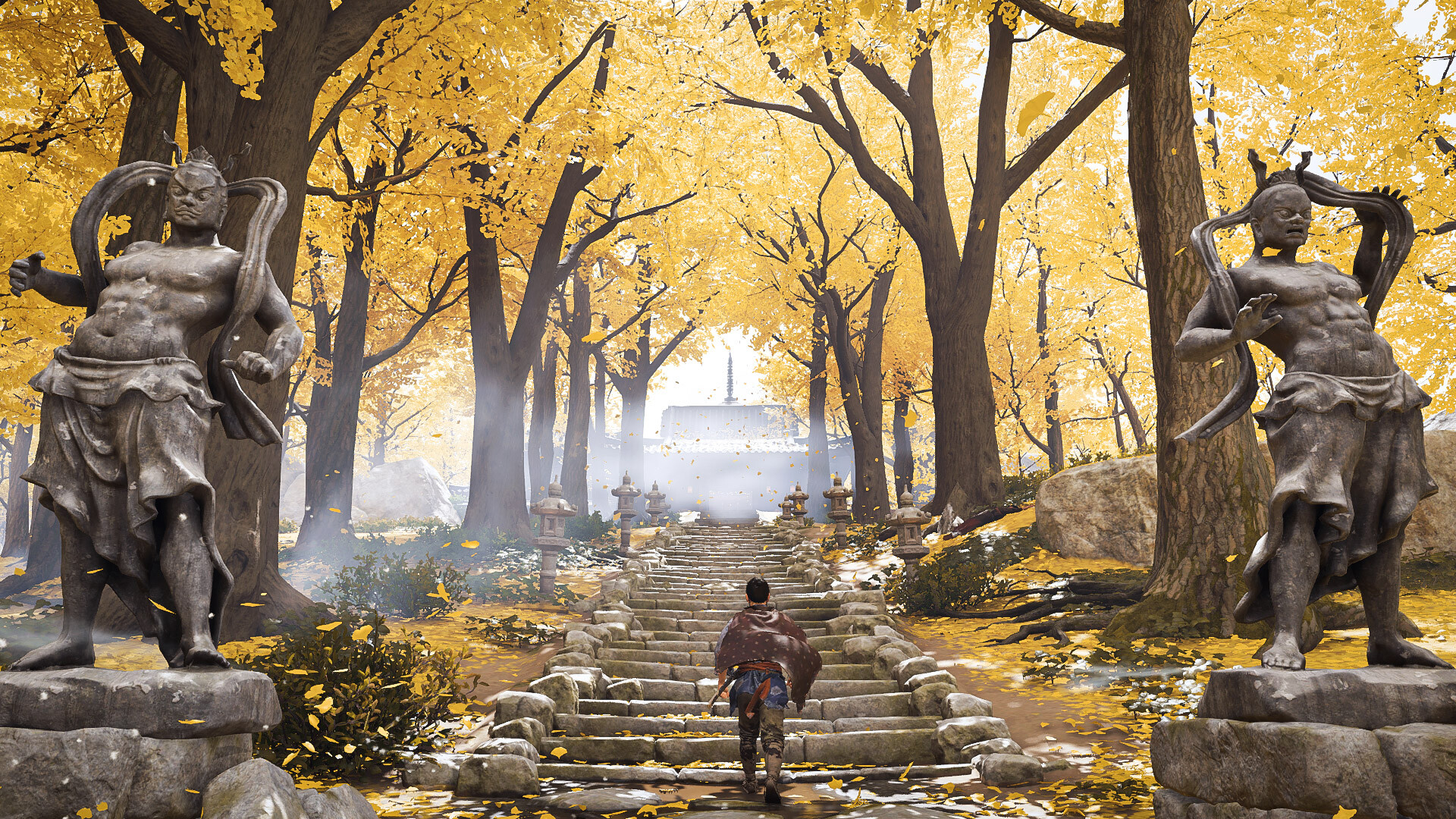The image depicts a mesmerizing horizontal rectangle scene that straddles the line between realism and surrealism. In the foreground, a row of wide, rock-concrete stairs, which narrow as they ascend, is framed by large rocks on either side. The weathered texture of the stones adds depth to the setting, guiding the viewer's eye upwards. At the top of the stairs, a structure, partially obscured by a haze of fog or smoke, invites curiosity while remaining mysterious.

Surrounding the stairway is a dense forest of trees with burnt-orange foliage and brown trunks that stretch upwards, casting a surreal, almost dreamlike atmosphere over the scene. The varying shades of orange contribute to the otherworldly impression of the forest.

Flanking the base of these stairs are statues of shirtless men draped in simple cloths and adorned with various items around their necks. Each stands proudly on a pedestal, adding an ancient and mythical quality to the image. In the midst of this enchanting setting, a lone man appears poised to ascend the stairs, his presence grounding the scene in a sense of impending journey or discovery.